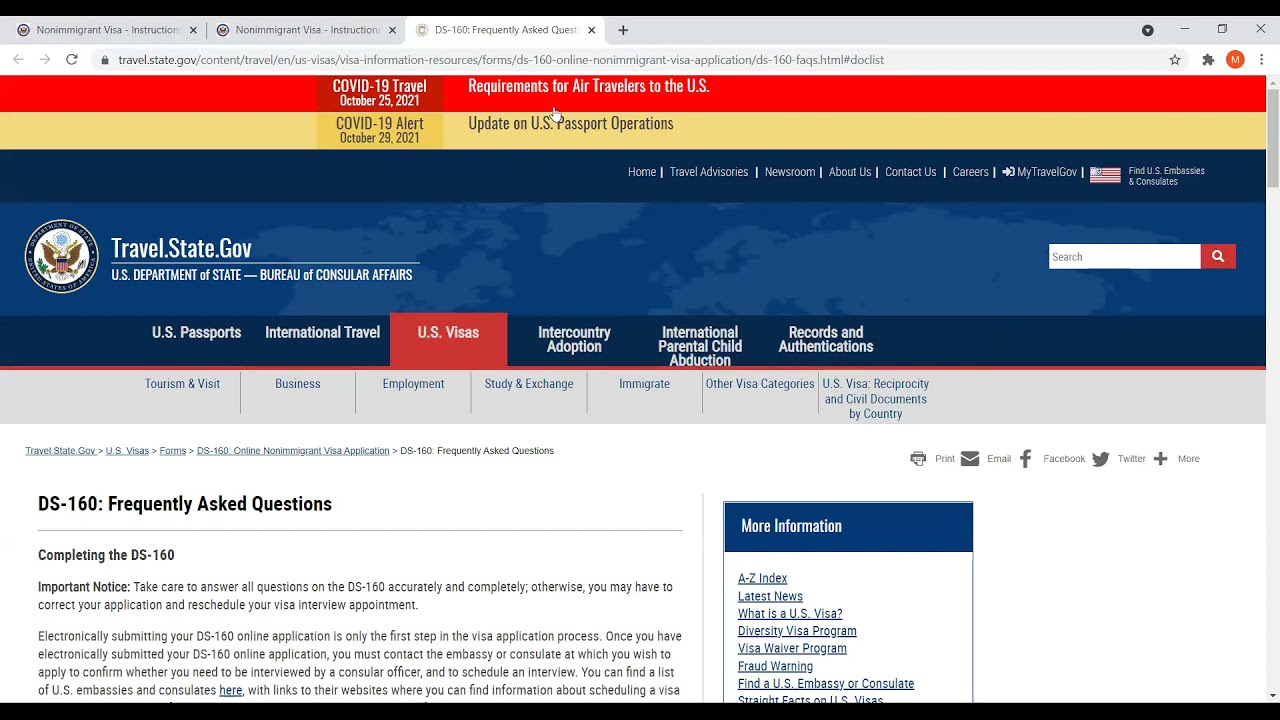Here's a detailed descriptive caption for the web page screenshot described:

---

The screenshot captures a multi-layered web page from the U.S. Department of State, specifically the Bureau of Consular Affairs. The foremost page prominently features a blue, gold, and red color scheme. The upper half of this page is predominantly blue, transitioning into a white background in the middle section where various text elements are displayed. The text includes headings such as "DS-160: Frequently Asked Questions" in bold black font, separated by a gray line. Additional details cover topics like "Completing the DS-160" and "Important Notice," advising users to carefully answer all questions.

On the right-hand side, a dark blue sidebar labeled "More Information" lists various links in white text, including "A to Z Index," "Latest News," and "What is the U.S. Visa." Directly above this sidebar, the interface features several icons representing an envelope, Facebook, Twitter, and a plus sign, presumably denoting options to email, share, or follow on social media. Further up, there are gray-text categories such as "Trip," "Tourism," "Visit," "Business," "Employment," "Study and Exchange," and "Immigrants," with some unreadable items in blue writing.

At the top part of the page, white text on the navigation bar includes sections like "U.S. Passports," "International Travel," "U.S. Visas," "Inter-country Adoption," "International Parental Child Abduction," and "Records and Authentications." An eagle emblem accompanies a "Travel State Gov" banner on the upper left side, representing the U.S. Department of State, Bureau of Consular Affairs. Adjacent to it, there is a white search box featuring a red square with a white magnifying glass icon.

The homepage navigation menu includes categories such as "Home," "Travel," and others, some partially obscured but likely including "About Us" and "Contact Us." Notably, a COVID-19 alert strip stands out in yellow, dated October 29, 2021, regarding updates on U.S. passport operations. Above this, another red banner dated October 25, 2021, details COVID-19 travel requirements for air travelers to the U.S. The entire page is framed within the general browser interface, identifiable by a gray "Travel State Gov" header and a search box featuring a star icon.